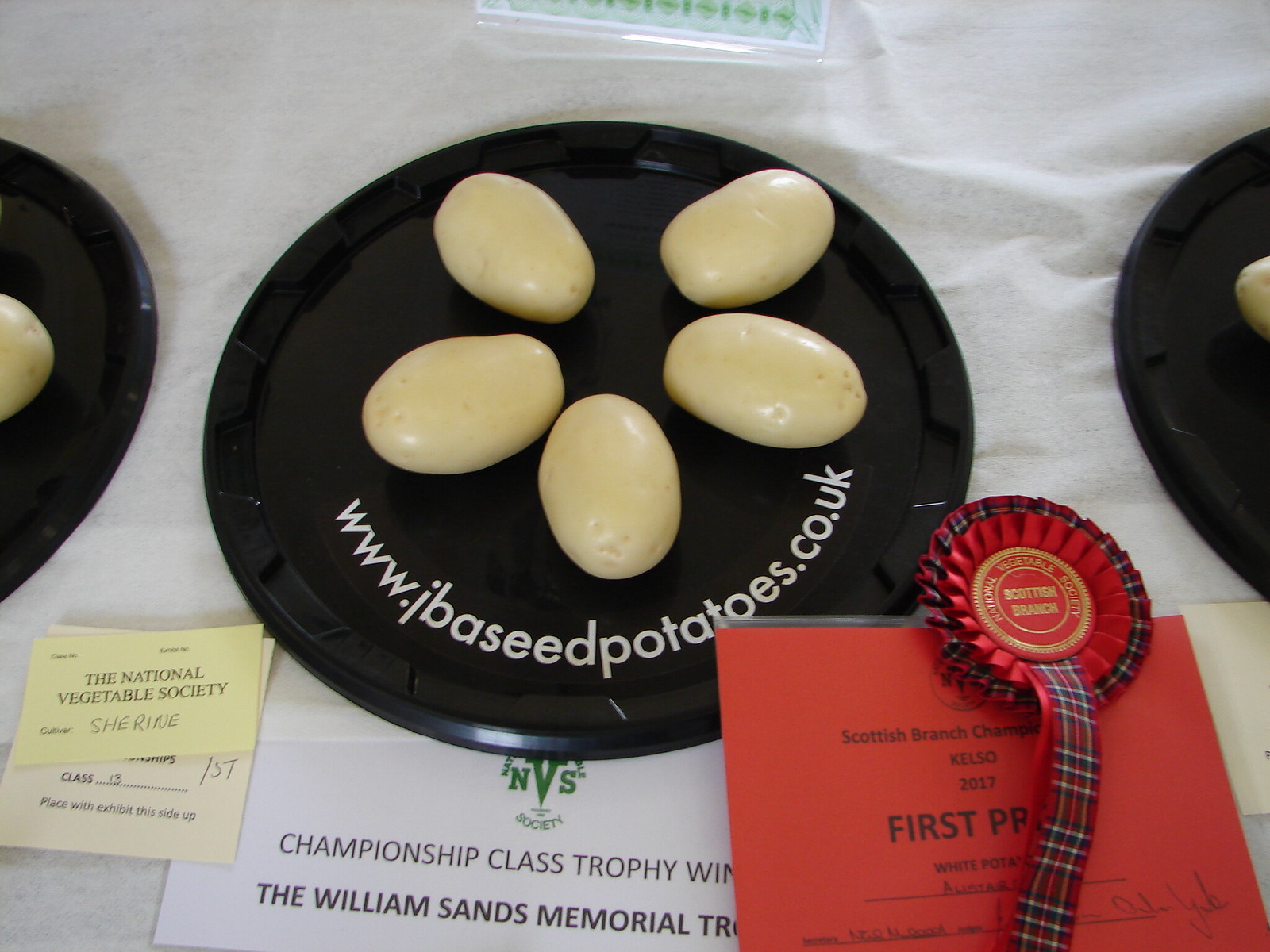The photograph captures a first prize-winning entry in a vegetable competition. Central to the image is a black plate, labeled with the website "www.jbayseedpotatoes.co.uk," bearing five small, light brown potatoes arranged in a circle. Flanking this central plate, there are partially visible identical plates with similar potato arrangements on both the left and right sides of the frame. Below the central plate, on the bottom left, there’s a note labeled "National Vegetable Society," with handwritten text reading "Shrine" and another note partially visible indicating "Class 13." To the right, a white paper announces "Championship Class Trophy Win" and "The William Sands Memorial Trophy," accompanied by a green "NBS" symbol. Further to the right, a red ribbon marked "Scottish Branch" is visible, along with a red paper underneath declaring "Scottish Branch Champion Kelso 2017 First Prize." The image is well-lit with natural light, highlighting the detailed and organized presentation of the competition entry.